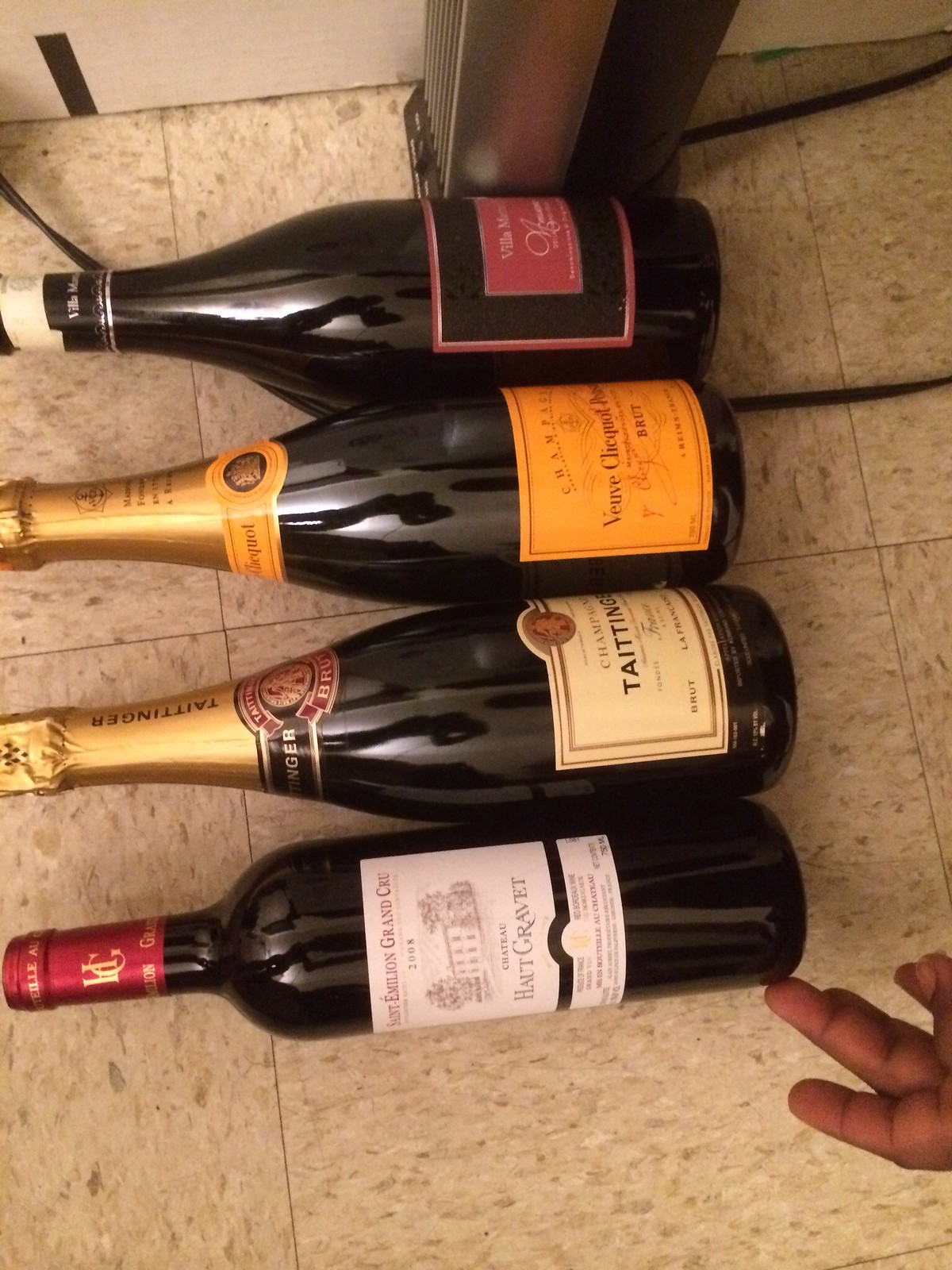The image shows four dark-colored wine bottles lying on an off-white speckled linoleum floor, all oriented with their corks pointing to the left and their bottoms to the right. The corks are pointing to a side angle, which makes the labels difficult to read. The first bottle, described as normal-sized, features a red and black label with a maroon cork cover and is slightly being touched by the ring fingertip of what appears to be an African-American man's left hand. The second bottle resembles a champagne bottle—it is fatter with a golden label at the top and an orange body. The third, about the same size, has a cream label with gold and black banding on the neck. The fourth bottle has a white label with black text and a red neck cover, with a hint of pink in the middle indicating the brand. Additionally, an electronic cord can be seen running over the top of the image, seemingly in contact with the first bottle.